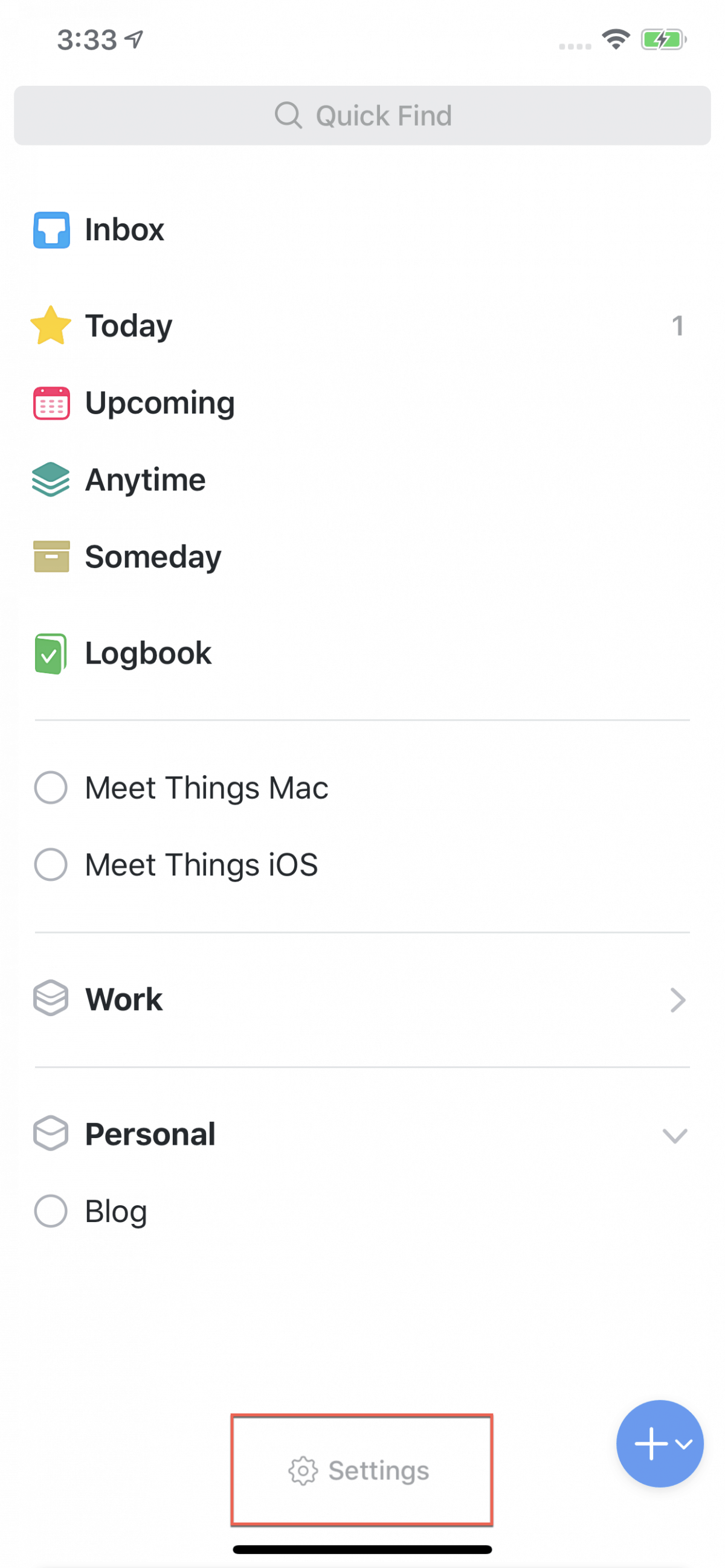Screenshot of a smartphone interface displaying a productivity app. The top of the screen shows a timestamp at 3:33, with a send icon on the far right. Next to the send icon are three vertical dots, a Wi-Fi icon, and a fully charged battery indicator. Below this is a grey search box featuring a magnifying glass icon and the text "Quick Find."

The interface includes vertical tabs on the left-hand side for navigation, labeled as: "Inbox," "Today," "Upcoming," "Anytime," "Someday," and "Logbook." There are selectable circles for different categories, such as "MeetThings Mac" and "MeetThings iOS."

Further down, there's a section labeled "Work" with a right-facing arrow on the far right. Below it is a "Personal" section that includes a drop-down arrow, potentially for more options under the blog category. 

At the very bottom, there is a settings box represented by a cog icon, alongside a blue circle featuring a plus sign with a drop-down arrow, likely for adding new items or tasks.